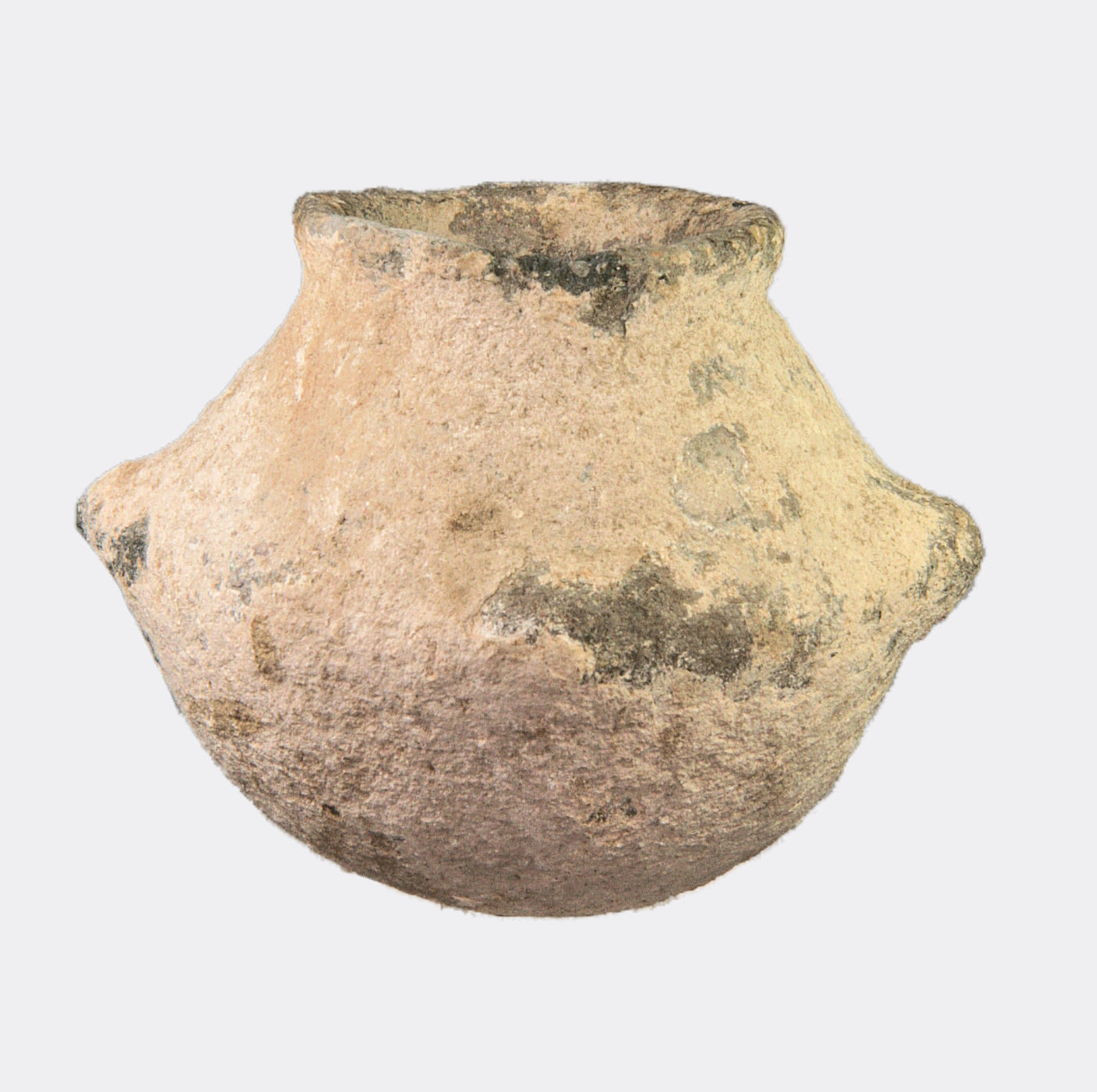The image is a photograph of a very old, possibly fossilized, pot or vase set against a blank light gray background, giving it a floating appearance. The pot is hand-carved from beige stone, featuring a rough, weathered surface dotted with various chips, nicks, cuts, and debris, indicating its age. The bottom is round, widening around the middle to facilitate carrying, then narrowing again towards the top, which opens into a circular rim. There are handles on either side of the pot, and its surface has darker, medium brown areas where the stone has chipped away, exposing a dirt-like color underneath. Triangular shapes jut out from the sides, adding to its ancient and rugged aesthetic.